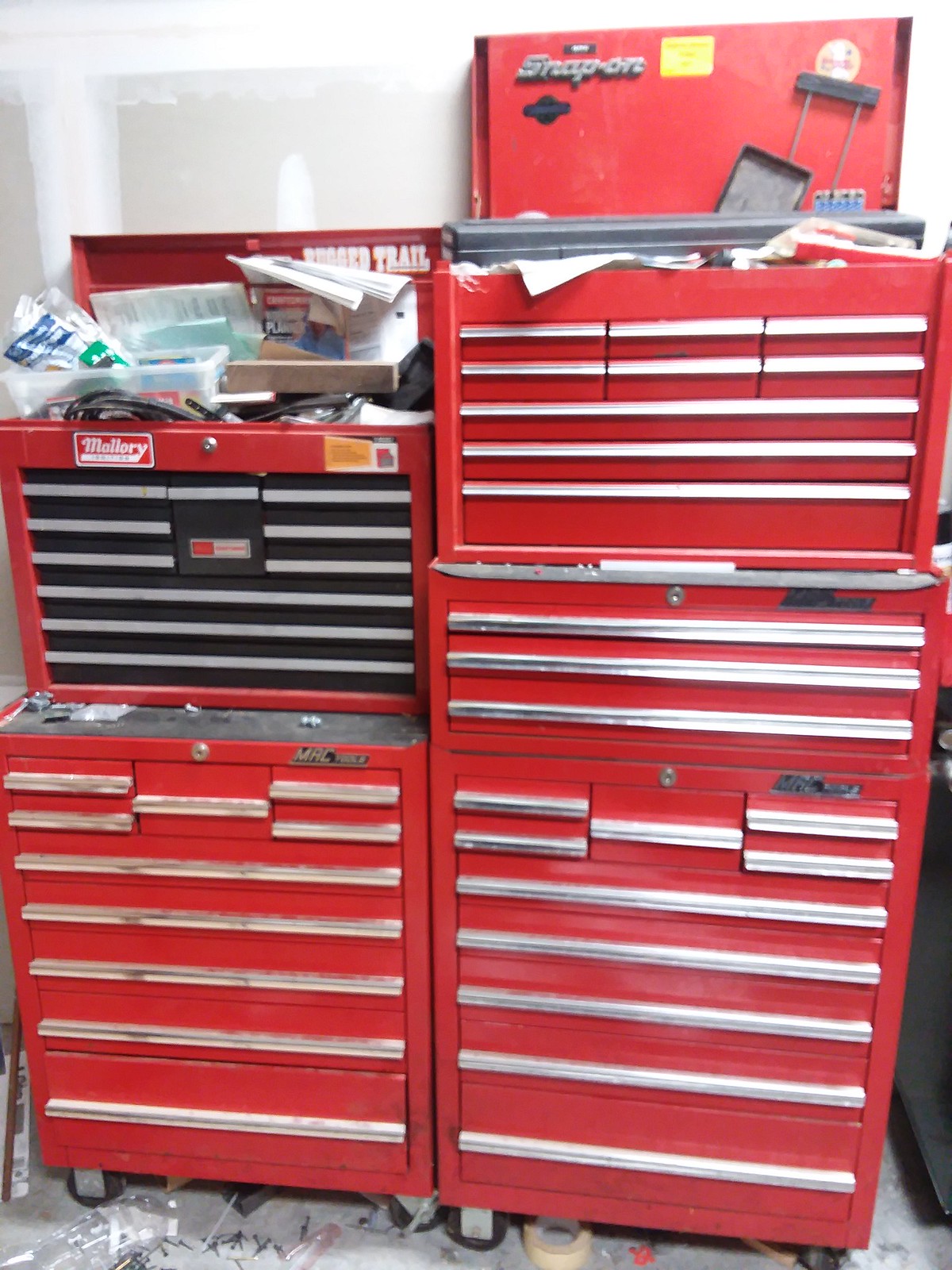The image showcases an extensive industrial-grade toolbox set, prominently red with silver handles and built on caster wheels for mobility. The setup includes two columns of tool chests, each with a series of drawers. The top two drawers in each column are open, revealing a mix of papers, plastic containers, and black wires. 

The toolbox in the upper left corner features a rounded rectangle emblem reading "Mallory" in white text on a red background, with smaller, unreadable text beneath it. This box's open lid partly reveals the words "rugged trail." Below it is another tool chest with drawers labeled "Mac something," likely "truck," which also appears on similar boxes in the lower left and right columns.

In the upper right, the toolbox lid seems to be branded "Snap-On" and contains black rectangular items and some red plastic parts among scattered papers. Surrounding the toolboxes, the floor is littered with assorted items such as a roll of tape, screws, and white plastic bits, all contributing to a dusty workspace. Despite the minor differences, the emphasis on the industrial, heavy-duty nature of these red enamel tool chests with their secure locking mechanisms and mixed drawer sizes is clear throughout the descriptions.